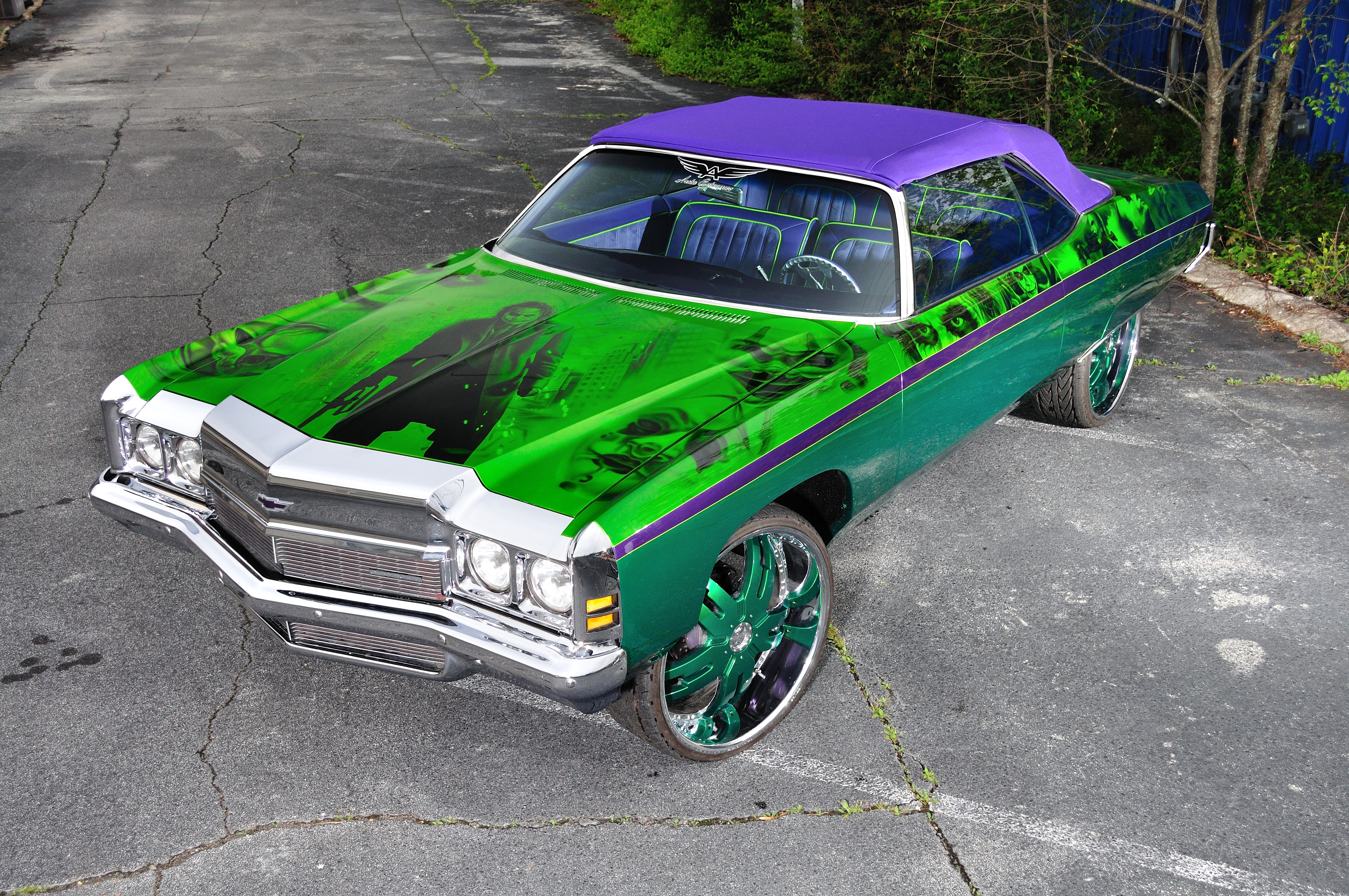In the image, an asphalt road, appearing weathered and worn with visible cracks and faded paint markings, serves as the ground floor. The road is flanked by patches of verdant grass and clusters of trees that provide a natural frame on both sides. At the center of the image, sharply contrasting the rugged backdrop, a silver car is diagonally parked, allowing a clear view of both its front and side. The setting is an outdoor parking lot, shrouded in nighttime dimness, which subtly highlights the car's metallic surface and the surrounding elements. The image palette comprises shades of gray, white, black, green, brown, silver, yellow, and a hint of purple, though no text is present to give further context. The composition positions the car as the focal point, reinforcing its prominence amidst the rugged road and natural borders.